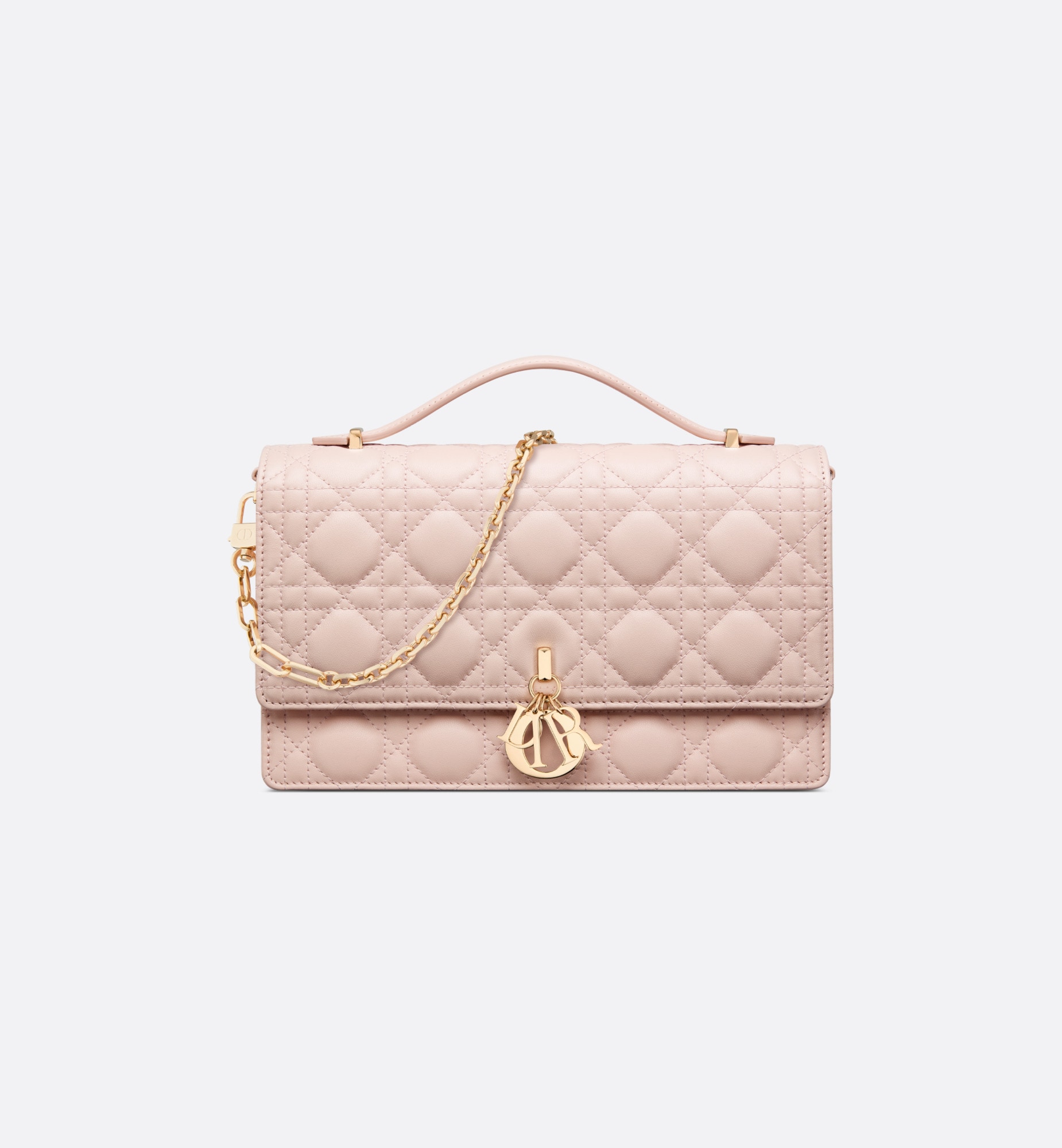The image features a luxurious, light pink quilted handbag with a refined aesthetic. The purse showcases an elegant geometric pattern, incorporating diamond shapes and circles crafted through meticulous stitching. It has an upside-down U-shaped pink handle, secured by gold buckles on either side, and a coordinating gold shoulder strap draped artfully over the top. The bag is slightly more substantial at the top, which folds over a slimmer bottom section, featuring a prominent gold clasp in the center. The clasp is adorned with the distinctive brand name "Dior," with the letters 'D', 'I', and 'R' dangling freely, while the 'O' is fixed, adding a sophisticated touch. The image is set against a pristine white background, emphasizing the purse's intricate details and upscale appearance.